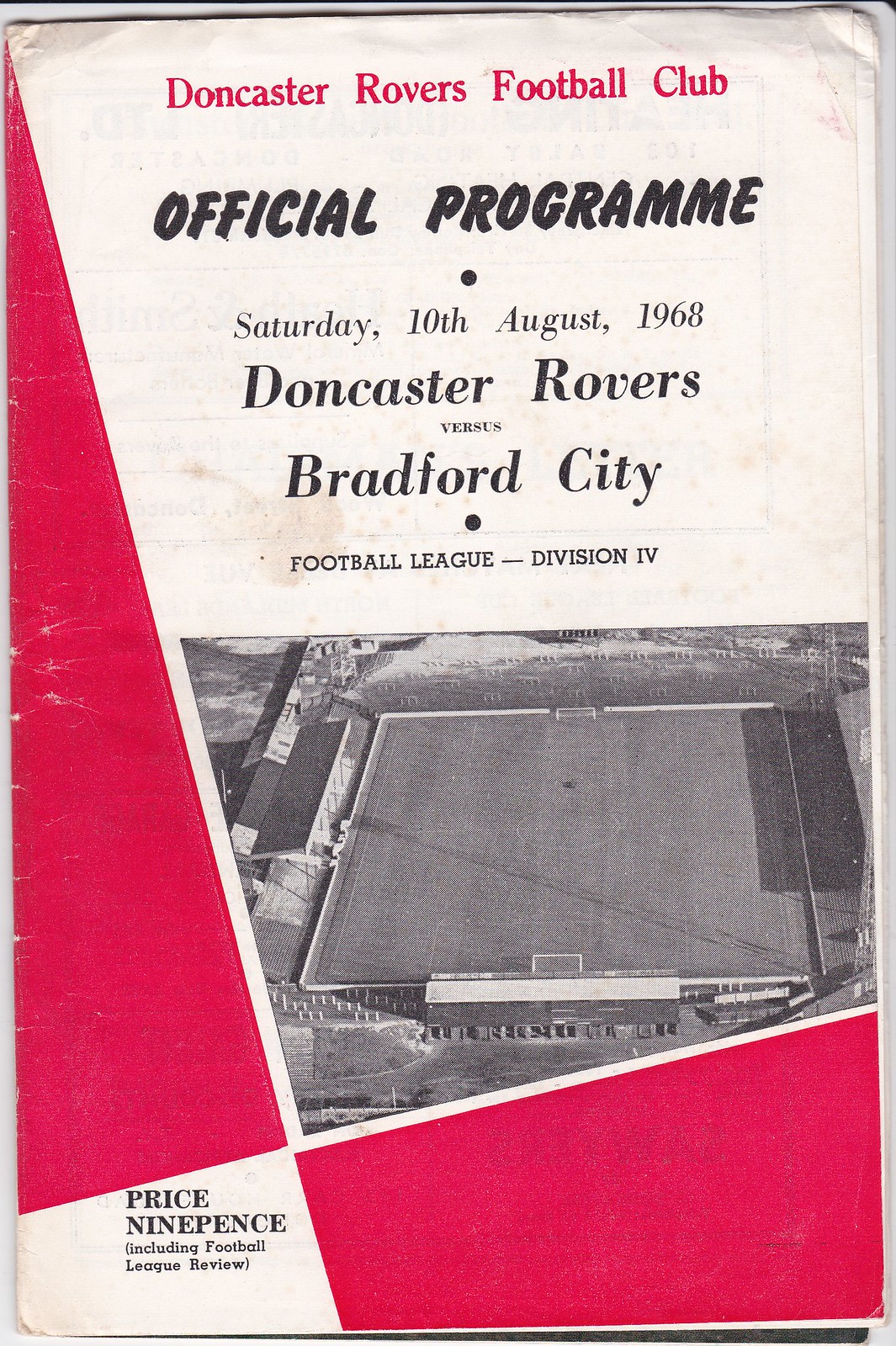This image showcases the aged cover of an official football program from Doncaster Rovers Football Club, dated Saturday, 10th August 1968. The yellowed paper features large red geometrical designs on the left side and bottom right corner, almost touching near the bottom center. The header is prominently marked in red with "Doncaster Rovers Football Club," followed by "Official Programme" in bold black text. Below the date, "Doncaster Rovers vs. Bradford City" is specified, along with "Football League Division IV" in Roman numerals. A black and white, pixelated image of an empty football stadium occupies the lower section. The program's price, "Price 9 Pence including Football League Review," is stated at the bottom left corner in black text. The overall condition hints at its age, showing slight stains and the impression of text from the next page.